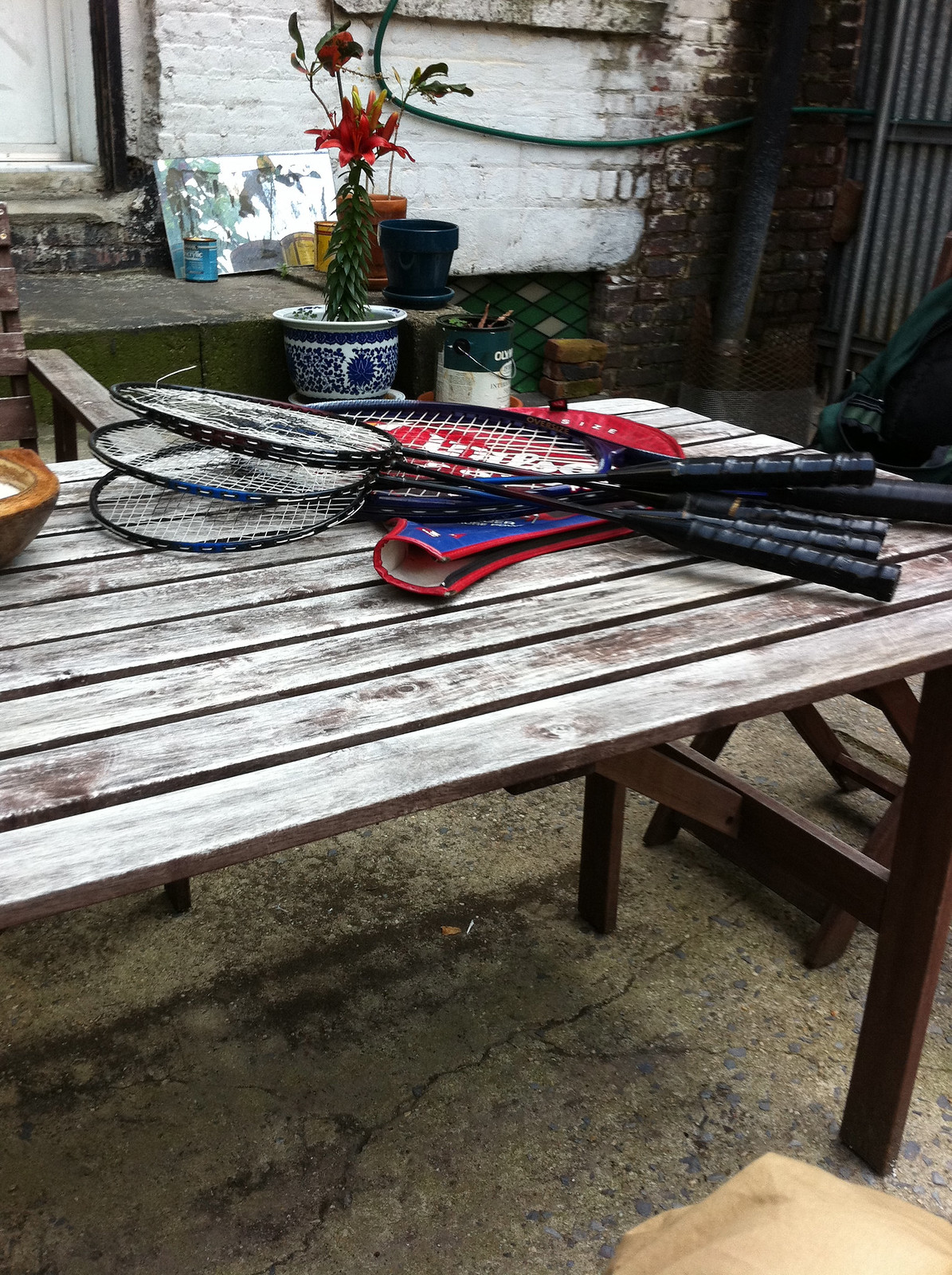This photograph depicts an outdoor scene in what appears to be a backyard patio area, featuring a weathered wooden table with faded, almost bleached, red paint. On top of the table is a collection of rackets, seemingly a mix of tennis and badminton rackets, identifiable by their narrow shafts and large black rubberized handles. These rackets, totaling around four, rest on a red and blue Wilson racket cover. The white webbing inside the heads of the rackets includes a distinctive black design.

Behind the table stands an old brick wall, partially painted white, with a section to the right where the paint has either flaked off or wasn't applied, revealing a dark red, almost burnt-looking surface. A black metal pipe runs along this section. Towards the upper left of the image, there's a white wooden door above concrete steps leading up. The steps and floor are both concrete, with the floor showing signs of age through cracks and discoloration from repeated wet exposure.

The patio area is adorned with various pots and plants. Notably, there's a striking white pot with a blue ornate design housing a lush green plant with a blossoming red flower. Nearby, a paint bucket repurposed as a planter sits amongst other flower pots. Also visible are items such as a small bowl on the table and potentially a chair under or behind the table, as well as potted plants along the wall, adding to the garden-like atmosphere of the space. The entire setting suggests an area that is both functional and in the midst of a simple renovation or cleaning effort, capturing a snapshot of a lived-in and loved backyard space.